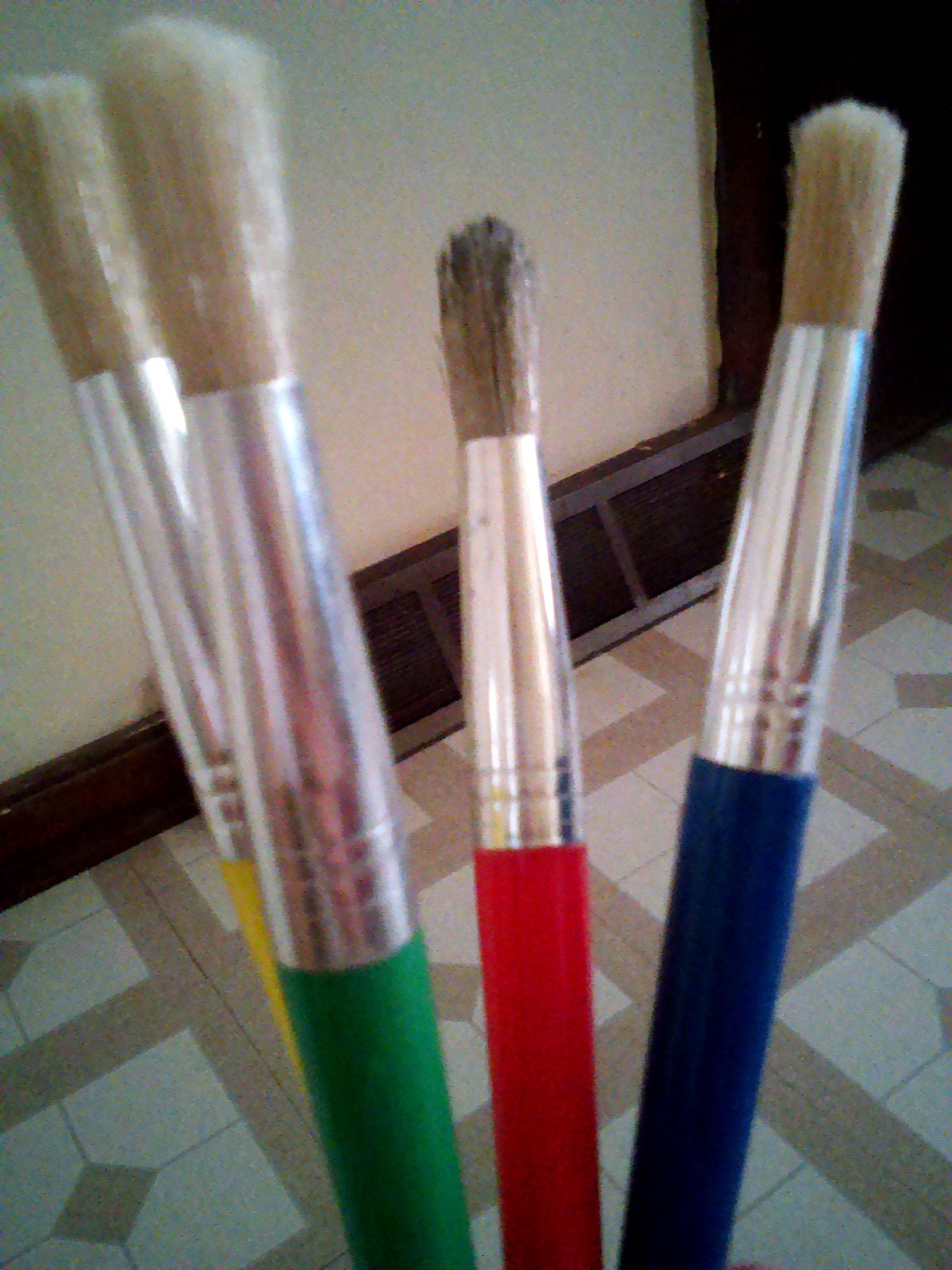This is a close-up photograph of four high-quality, bulbous, round-tipped artists' brushes, each featuring a silver ferrule. The brushes are held up so we can see their colored handles and white bristles clearly. The handles are painted in distinct colors: yellow, green, red, and blue. Notably, the red-handled brush appears slightly soiled with what seems like dark-colored, possibly bluish or reddish, paint, whereas the other three brushes look clean and unused. The background reveals a tile floor with tan and ivory hues and a baseboard leading up to light gray or white walls. A black return air vent situated to the right is slightly tilted, adding a touch of character to the setting. The perspective provides a downward view, making it evident that the brushes are held at floor level.